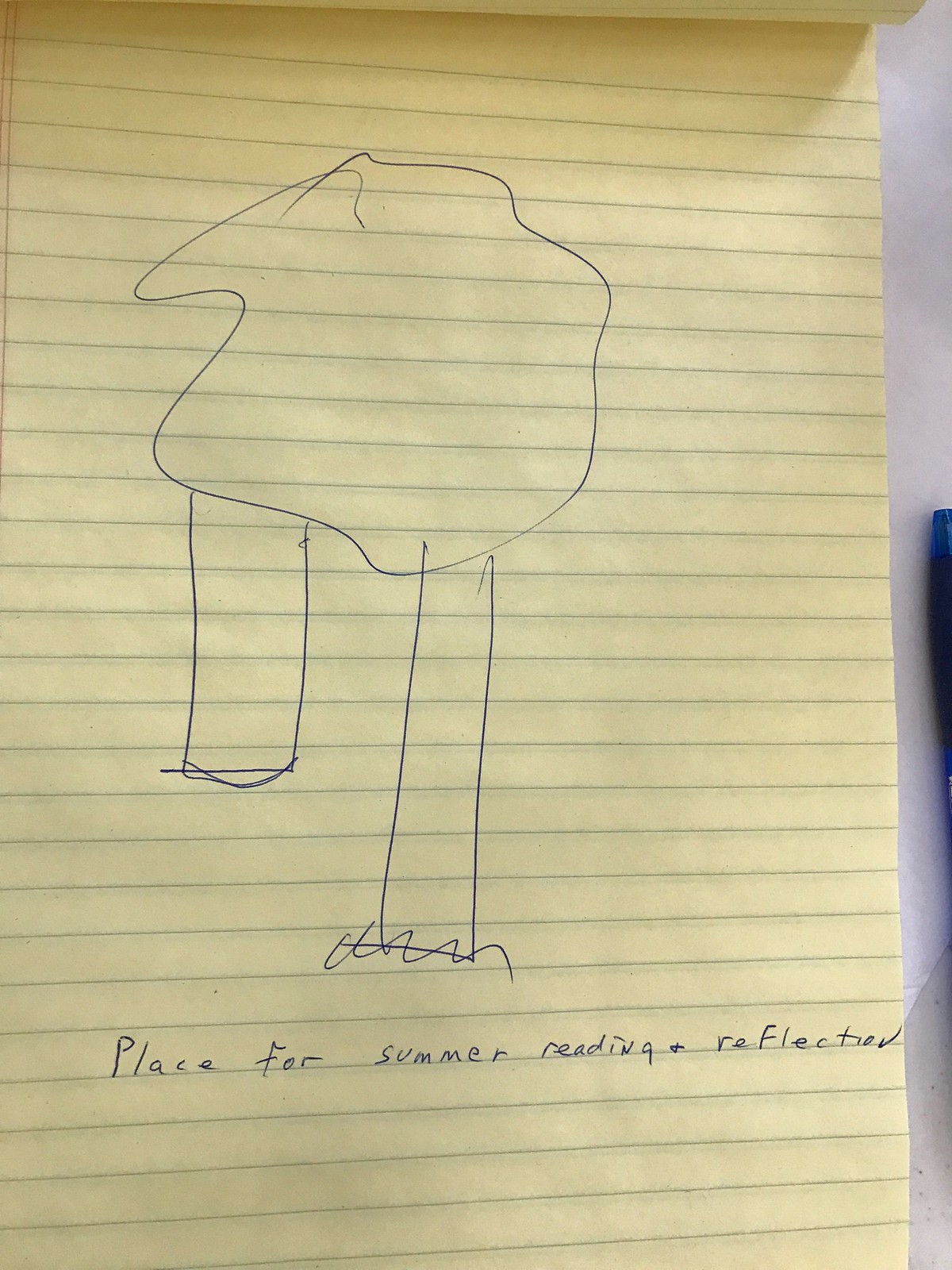This image features a rough sketch drawn on an 8.5 by 11 inch yellow lined notepad. The sketch, rendered in blue ink, depicts what appears to be two tree-like structures sharing a single canopy of leaves. Alternatively, the drawing could be conceptualizing a structural design, resembling two columns of differing lengths, with the nearer column being longer, possibly to suggest perspective or dimension. The canopy atop these columns has an abstract shape: the left side forms what looks like a cursive letter "E," while the right side features a protrusion resembling a nose, though the overall form is quite amorphous. Below the sketch, a handwritten note in blue ink reads, "Place for Summer Reading and Reflection," hinting at the purpose or inspiration behind the design.